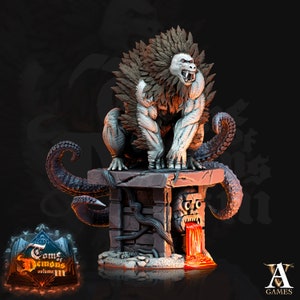The image depicts a dark, black background with a prominently detailed 3D figurine. The main subject is a fierce, hybrid creature perched on a gray, Aztec-inspired stone pedestal. The creature has a body resembling that of a gorilla, with thick muscles, prominent sharp fangs, and a menacing face. Its head features the mane of a lion while tentacles, akin to those of an octopus, extend from its back, adding to its nightmarish appearance.

The pedestal, appearing either stone or wooden, has a tribal face carved on its side. The eyes are wide open, and the mouth is agape with fiery or red lava-like substance pouring out. The overall mood of the scene is ominous and unsettling.

In the bottom left-hand corner, text reads "Tome of Demons Vol 3," with "Tome" in white and "Demons Vol 3" in fiery orange text. The bottom right-hand corner contains the logo "VA Games" or "AV Games" with a distinctive large white "A" against a brass "V." The image also contains a watermark which is not clearly defined. The overall illustration evokes a sense of dread and fantasy, possibly related to a game.